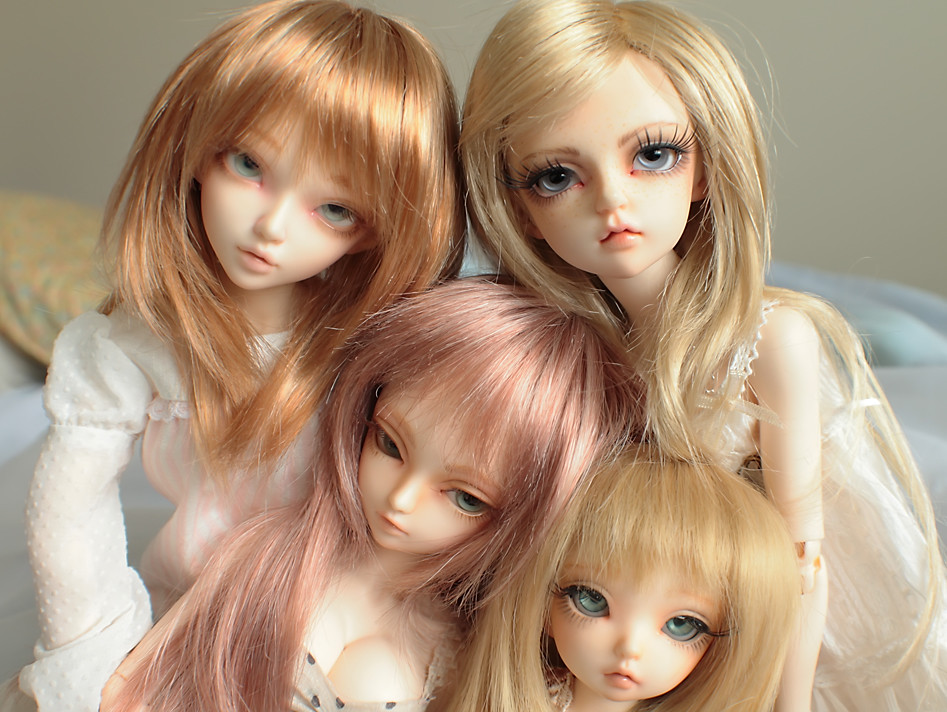This image showcases a collection of four visually striking dolls, each exhibiting unique features and variations. These dolls possess pale, intricately detailed faces and wear white, frilly, gauzy attire that gives them an ethereal and somewhat unsettling appearance. Their large, blue, anime-like eyes are accentuated by exceptionally long and dark eyelashes, the longest belonging to the doll on the far right. Each doll has a distinct hair color—ranging from pale blonde to ginger and blush. The ginger-haired doll sports bangs, adding to the individuality of each figure. Among them, the doll with blush hair stands out with her prominent bustline, heavily emphasizing the adult and sultry design of these dolls. Two smaller dolls are nestled near the bottom; one has pink hair, and the other, partially visible with a youthful appearance, has blonde hair. The backdrop of the scene features a grayish-green wall and some blankets, contributing to the overall beige tone of the image. The dolls, with their pouting big lips, and highly sexualized expressions, evoke an almost eerie, otherworldly presence.